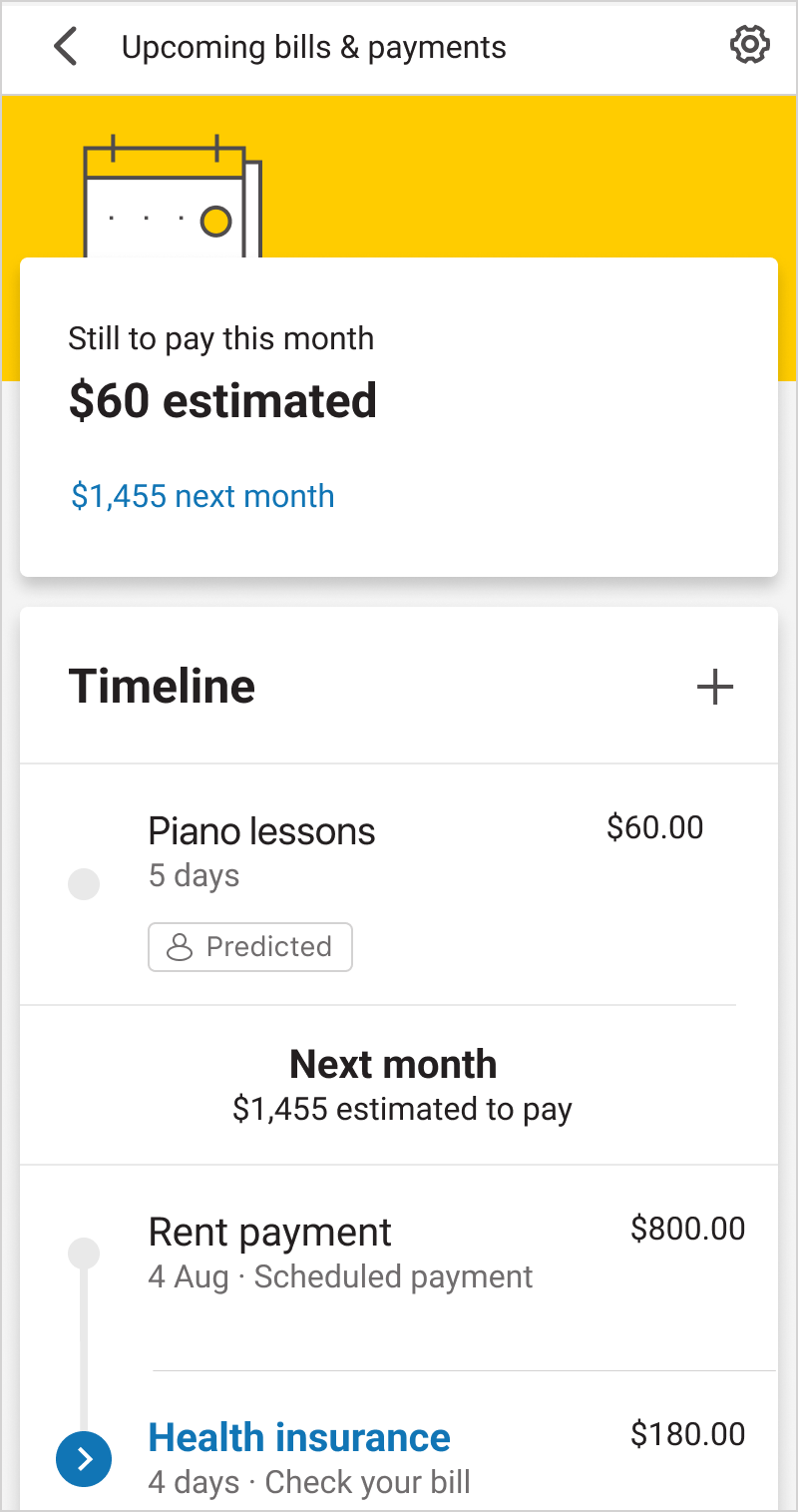The screenshot showcases the interface of a smartphone app displaying upcoming bills and payments. At the top left, a left-facing arrow is visible, followed by the heading "Upcoming Bills and Payments." A gear icon appears in the upper right corner, suggesting settings or configuration options.

Highlighted in blue, there is a reminder: "$1,455 next month." Beneath this, the text in black reads, "Estimated to pay this month: $60." A timeline of expenses is detailed below, beginning with "Piano lessons: $60," marked five days from now in black text. Indented further, a summary of the next month's estimated amount due is repeated: "$1,455."

At the bottom of this timeline, several specific payments are listed in black text, including "Rent payment: $800 scheduled for August 4th" and "Health insurance: $180," which is due in four days and marked for verification with a dot noting "Check your bill." The health insurance payment is highlighted in blue and there is a right arrow suggesting more options or details.

The top section of the screen features a yellow background with a cute robot avatar design, adding a playful touch to the otherwise functional interface. This detailed view organizes upcoming financial commitments into clear, accessible categories on a smartphone screen, aiding users in keeping track of their monthly expenses.